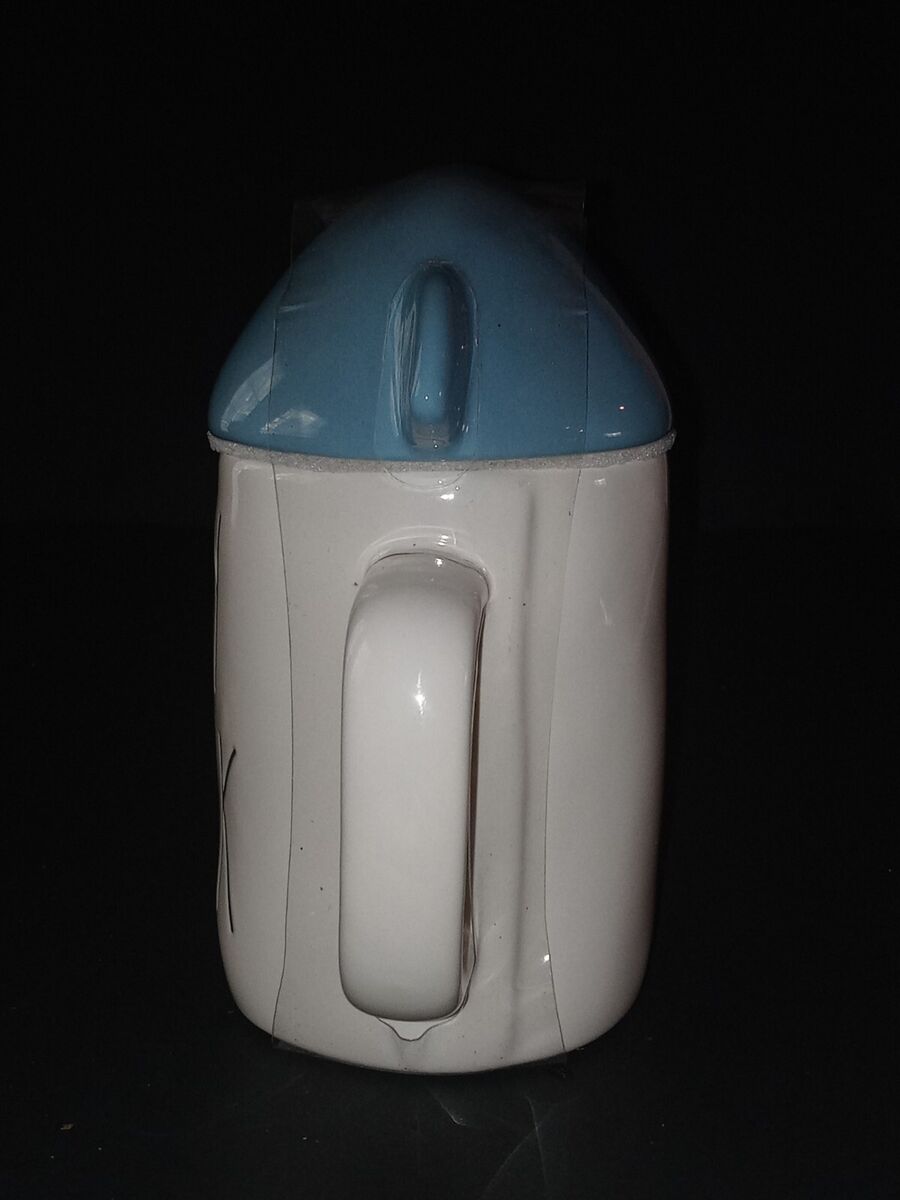The image showcases a white, glossy ceramic mug with a large, prominently facing handle, reminiscent of a coffee mug or creamer pitcher. The mug is topped with a dome-shaped blue ceramic lid, which features a small tab for easy removal. The lid and the mug are secured together by a plastic strap, suggesting it might be a new product. The left side of the mug appears to have some form of etching or engraving, though details are obscured from view. The setting includes a black background with a light source, likely a flash, casting reflections on the mug's surface, emphasizing its glossy finish. The photograph's angle and lighting hint at it being part of a series, possibly for an online listing, where multiple perspectives are provided.